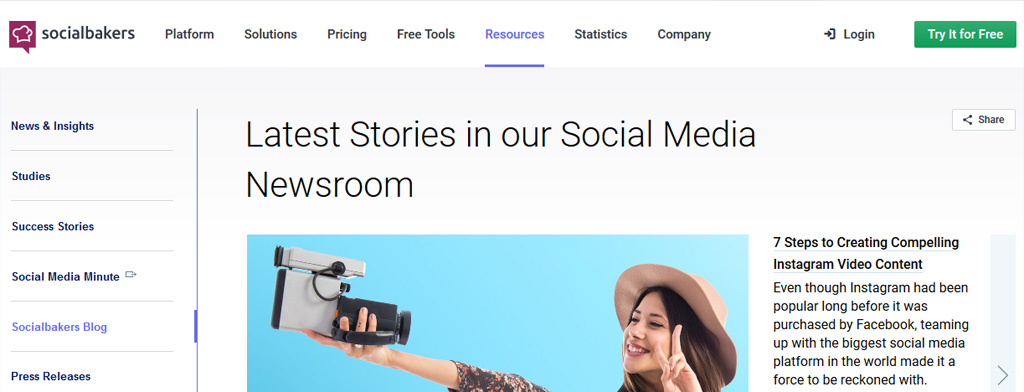This is a detailed and descriptive caption for the given image:

"The image is a horizontal rectangular snapshot of a web page belonging to Social Bakers. In the top left corner, the Social Bakers logo is displayed prominently in all lowercase black letters, accompanied by a magenta dialog box icon featuring a white chef's hat. Heading from left to right across the top navigation bar, categories listed in small black font include 'Platform,' 'Solutions,' 'Pricing,' 'Free Tools,' 'Resources'—the latter distinguished by a blue-purple font with an underline. Continuing to the right, subsequent categories are 'Statistics' and 'Company' in black font, followed by 'Login,' and a prominent green rectangular button with white text reading 'Try It For Free.'

At the center of the image, a bold black font headline states, 'Latest Stories in our Social Media Newsroom,' with 'Latest Stories,' 'Social Media,' and 'Newsroom' capitalized. Below this, a horizontal rectangular image with a turquoise background depicts a woman wearing a light brown cowboy shirt. She is holding up a peace sign with her left hand while taking a selfie with a camera in her extended right hand. To the right of this image, in bold black lettering, is the title, '7 Steps to Creating Compelling Instagram Video Content.' Below this title, in standard black font, is a brief paragraph: 'Even though Instagram had been popular long before it was purchased by Facebook, teaming up with the biggest social media platform in the world made it a force to be reckoned with.'

Along the left side of the web page is a navigation column featuring categories labeled 'News and Insights,' 'Studies,' 'Success Stories,' 'Social Media Minute,' 'Social Bakers Blog'—highlighted in purple—and 'Press Release.'"